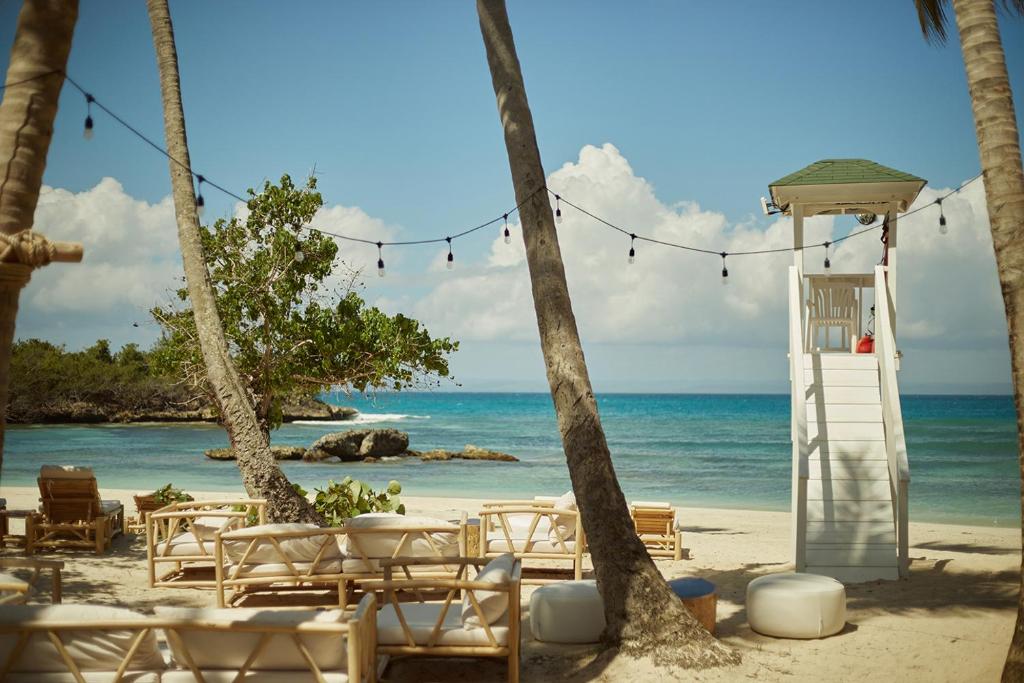This photograph captures a stunning beach setting bathed in daylight. In the foreground, a pristine sandy white beach extends out, adorned with beach furniture made of light blonde wood and off-white cushions. Numerous trees with light brown trunks dot the landscape, adding a rustic charm. A white lifeguard station with a green roof stands prominently, featuring a white chair ready for the lifeguard's duty. Strung between the trees is a whimsical string of black lights with white bulbs. The turquoise ocean stretches out in the middle ground, with rock formations rising from the water, and a rock outcropping adorned with green shrubbery off to the side. The scene is completed by a clear blue sky dotted with fluffy white clouds, making it a perfect beach day.